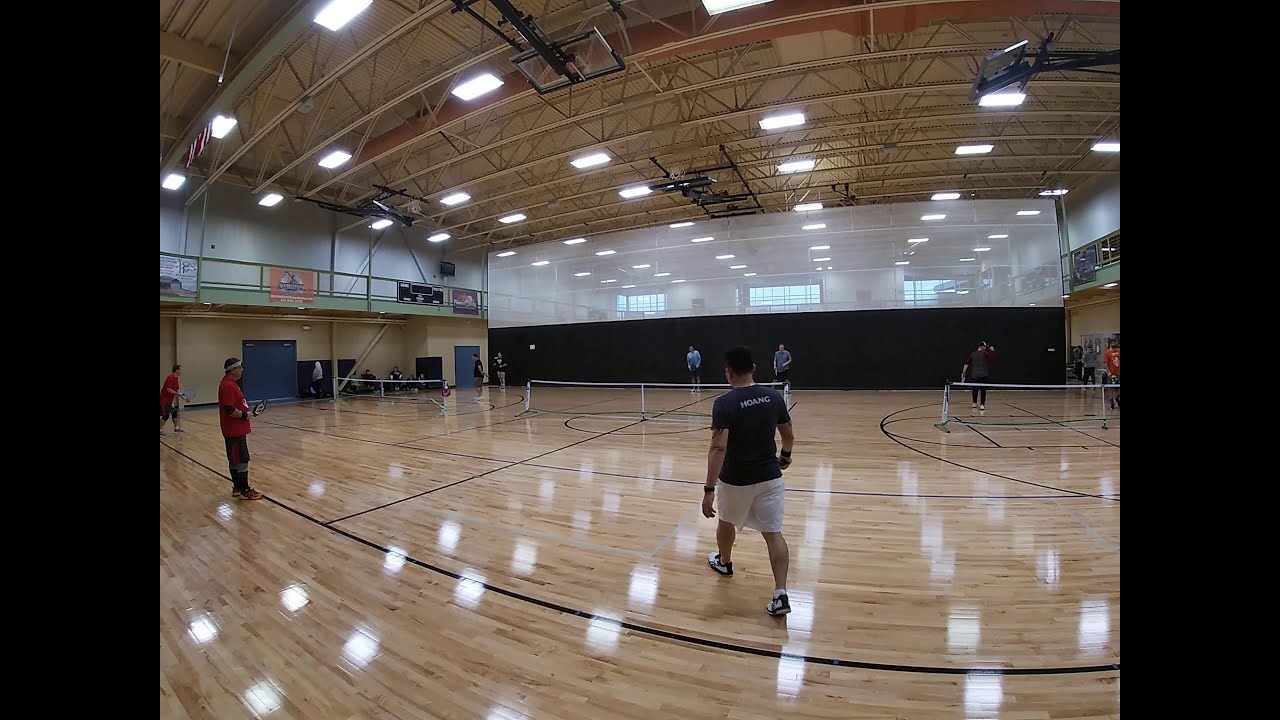The image depicts an indoor sports complex with a polished hardwood floor that reflects the numerous fluorescent lights overhead. The area is currently set up for multiple games, with three white and black tennis nets installed across the floor. Various black lines and circles are painted on the brown flooring to indicate different play areas. The high ceiling, supported by steel beams, is mostly tan and white in color with rectangular fluorescent lights illuminating the room. Basketball hoops are folded up toward the ceiling to accommodate the tennis setup. The setting includes people dressed in athletic gear—shorts, sweatpants, elbow pads, headbands, and athletic shoes—engaged in active play. The walls of the complex are plain white, and there is a visible divider in the middle of the room, further segmenting the playing area.